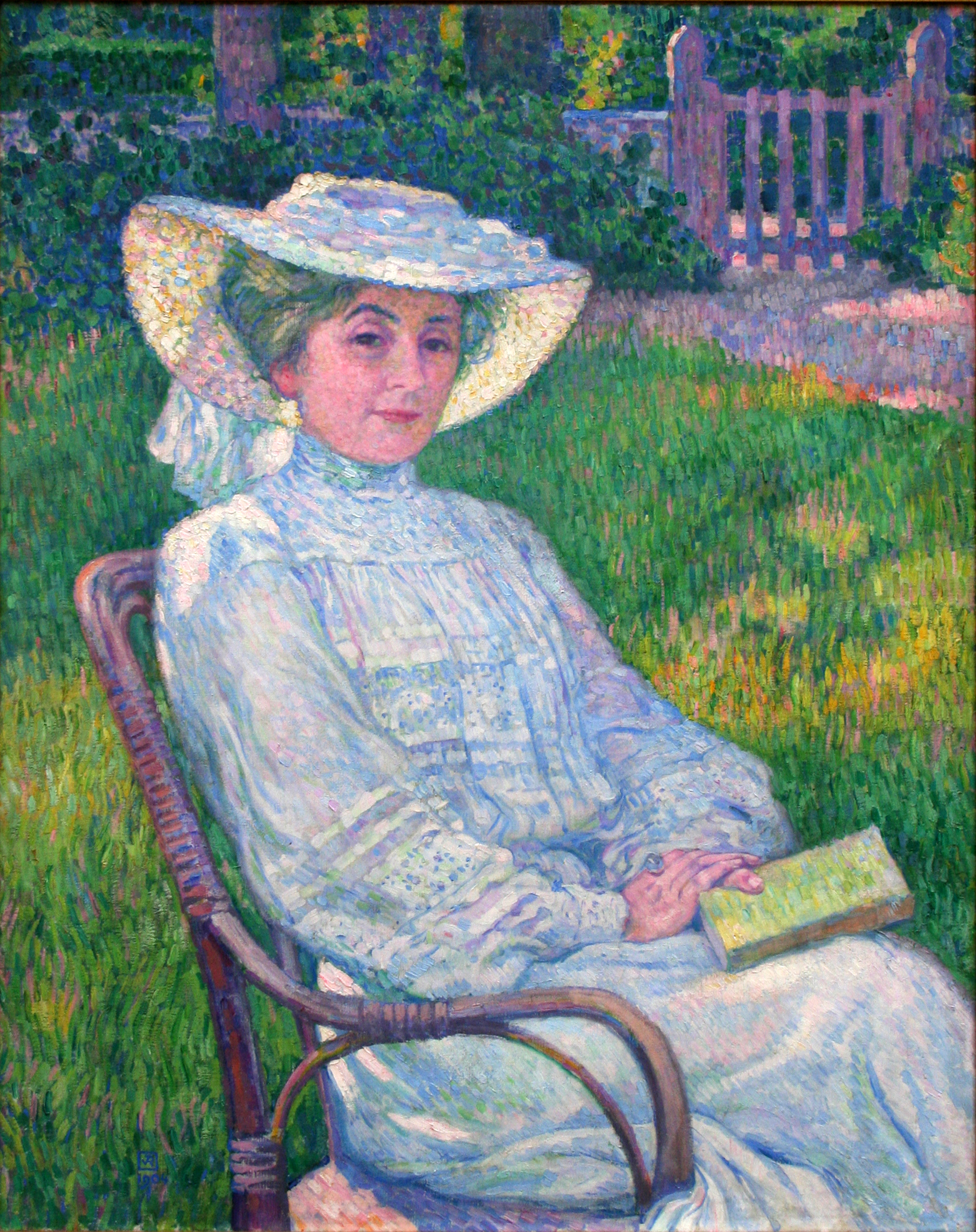The painting depicts a woman in her late 50s to early 60s, sitting in a wooden chair in a well-manicured garden, possibly her front yard. She's dressed in a white sun hat and a white sundress adorned with hints of faded red and blue, which extends up to a collar around her neck. Her hair, with a greenish tint and streaks of brown and gray, peeks from under her hat. She wears a blue ring on her index finger. The woman has a serene, satisfied expression with bright eyes and a soft smile. She's holding a green book with her hands gently clasping it. Surrounding the garden are lush green and yellow-tinted grass, suggesting varied sunlight. Behind her, there's a purple-painted fence gate with ivy climbing on it, flanked by tree trunks and foliage, leading in from a visible pathway. To the left of the scene, flowers add a touch of color. The overall style of the painting combines elements reminiscent of both Rembrandt and Impressionist art, capturing a peaceful, reflective moment on a summer day.